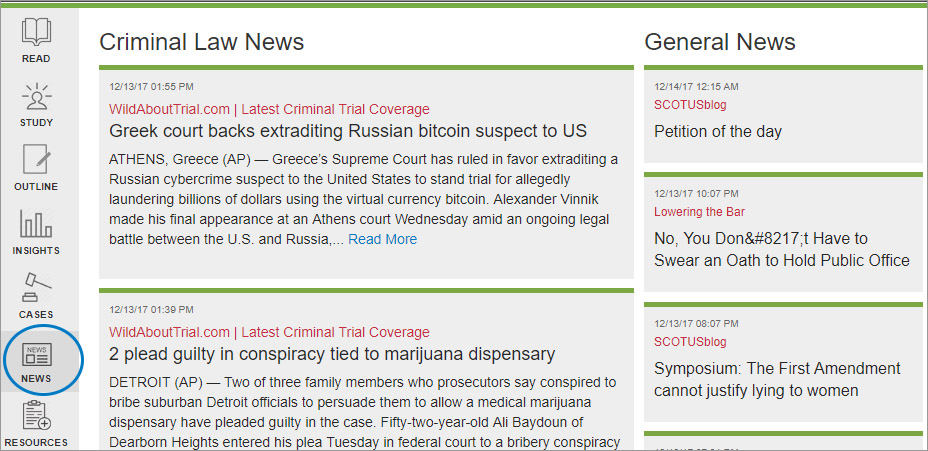In this image set against a white and gray background, a navigation bar is visible on the left side, featuring various icons and labels: a book icon labeled "Read," a human body icon labeled "Study," a paper and pencil icon labeled "Outline," icons for "Insights," "Cases," and "News" with a blue circle, and a "Resources" section. 

On the upper right in large text, it reads "Criminal Law News." Below this heading, in red text, is the timestamp "12.13.2017 1:55 p.m." followed by the source "wildabouttrial.com" and the tagline "Latest Criminal Trial Coverage." 

Further down, the main headline in black text states: "Greek court backs extraditing Russian Bitcoin suspect to US." The accompanying subtext reads: "Athens, Greece (AP) — Greece's Supreme Court has ruled in favor of extraditing a Russian cybercrime suspect to the United States to stand trial for allegedly laundering billions of dollars through the virtual currency Bitcoin."